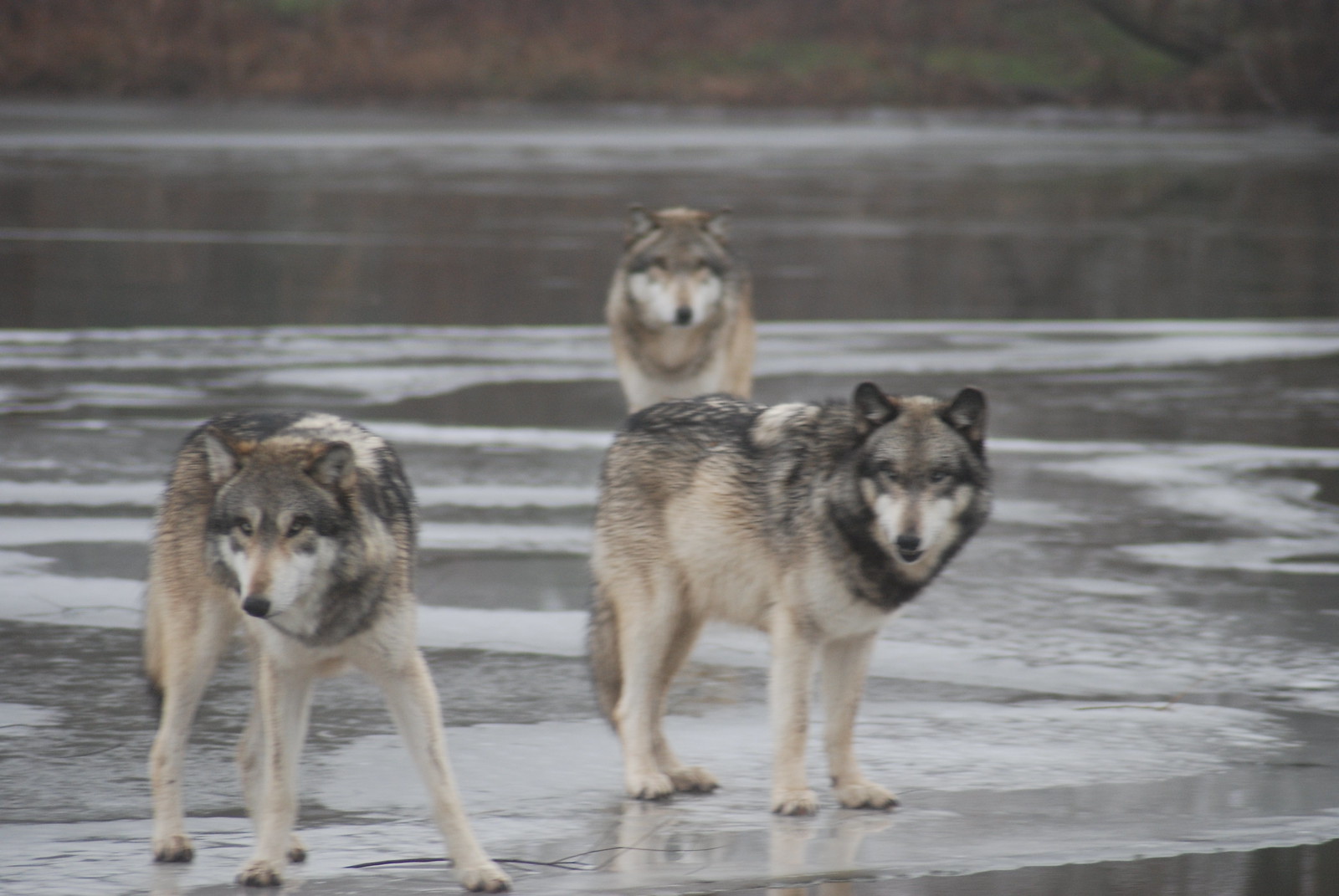In this detailed outdoor photo, three wolves stand on a frozen lake under daylight, facing in the direction of the camera but not directly at it. The two wolves nearest the camera exhibit a blend of darker colors, including black, brown, and gray, while the wolf in the background possesses a lighter coat with shades of dark gray and tan. The ice beneath them glistens, revealing a stick frozen in place. The landscape-oriented image captures a transitional scene where the ice-covered lake meets the water in the background, framed by a distant hillside and trees. The wolves, slightly wary and alert to something off-frame, embody the wild spirit of their natural habitat.